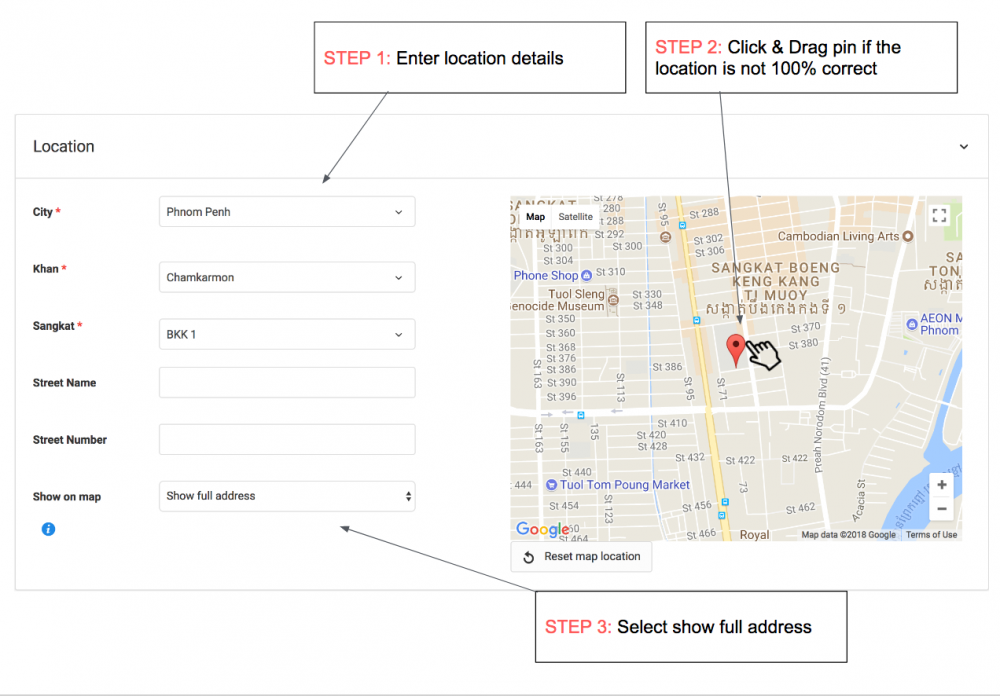This image displays a detailed interface of a location-finding tool utilizing Google Maps. At the top, there are two adjacent blocks labeled "Step 1: Enter location details." Step one encourages users to enter the necessary details about their location, whereas step two instructs users to click and drag the pin if the location is not accurate. The left side features a list of search options with dropdown menus for specifying the city (con, written as K-H-A-N), followed by S-A-N-G-K-A-T, street name, and street number. Additional options include buttons to "Show on map" and "Show full address."

On the right side of the interface, there is a visual representation of a Google Map, showing a detailed map with a prominent red location pin in the center. Accompanying the pin is a cursor hand icon, suggesting interactivity. The map exemplifies an oriental geographic region. Below the map, a square marked "Step 3: Select show full address" is illustrated with an arrow pointing back to the location search options.

The map interface also includes an option to "Reset map location," allowing users to correct any misplacements easily. This robust interface assists users in accurately pinpointing and displaying comprehensive location information on the map.